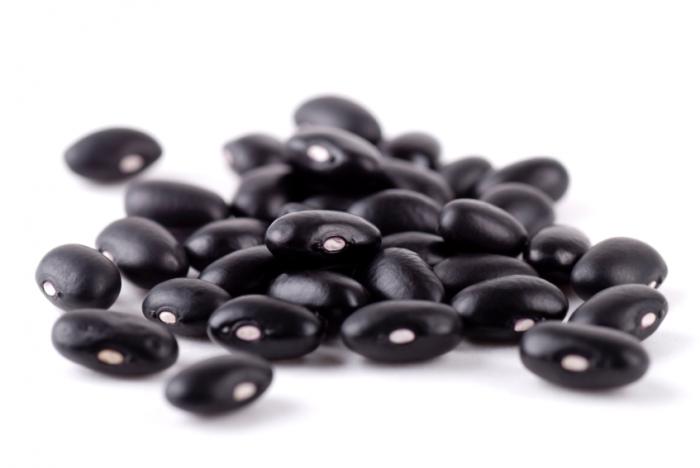The image depicts approximately 30 to 40 dried black beans clustered on a plain white surface, likely a table or dish, as suggested by the shadows each bean casts. The beans are predominantly in a single layer, although a few lie atop others, creating a small, uneven pile. Each bean is characterized by small white spots or inlets, typical of black beans. The image has a sharp focus in the center, with a slightly blurry periphery, emphasizing the textured details of the beans and their shadows against the stark white background.